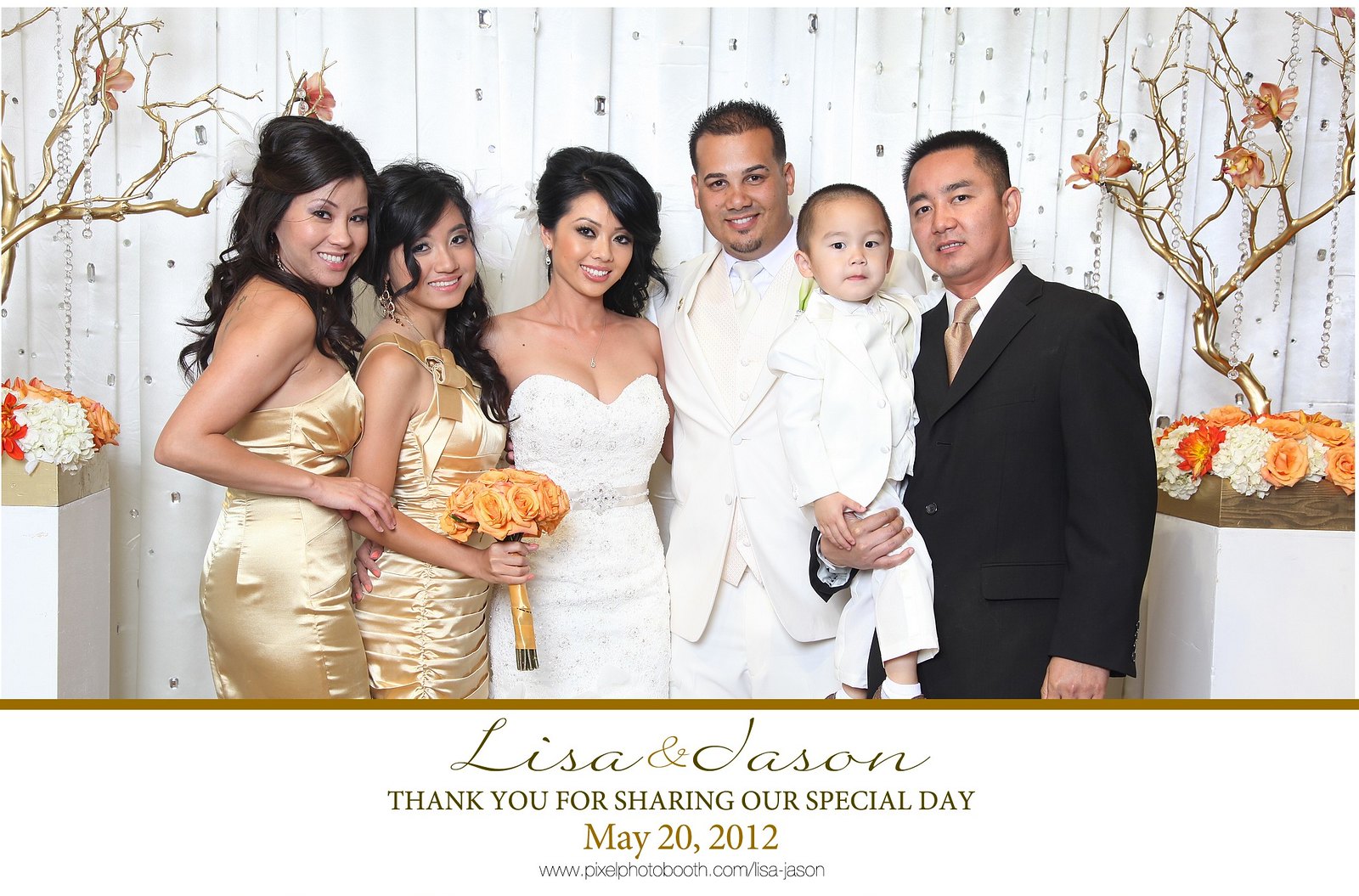In this detailed wedding thank you card, the centerpiece is a photograph showcasing six people. The bride and groom are central to the image; the bride wears a long, elegant white dress, while the groom complements her in a white suit jacket, an unusually stylish choice befitting the joyous occasion. The bride is flanked by two bridesmaids in shimmering gold dresses, situated to her left. To the groom's right stands a groomsman, dressed in a black suit jacket and a gold tie, holding a child. They are all posing against a backdrop featuring decorative elements: tall, fancy golden trees adorned with red, yellow, and white blossoms, positioned symmetrically on either side. Behind them is a neutral wall that enhances the atmospheric composition. Below this heartwarming image, there is a note rendered with elegant cursive and all-capital text, respectively, which reads: "Lisa and Jason, thank you for sharing our special day, May 20th, 2022." Accompanying this is the URL www.pixelfotobooth.com/LisaJason. The entire scene captures the essence of a beautiful celebration and serves as a cherished memento from the couple to their guests.